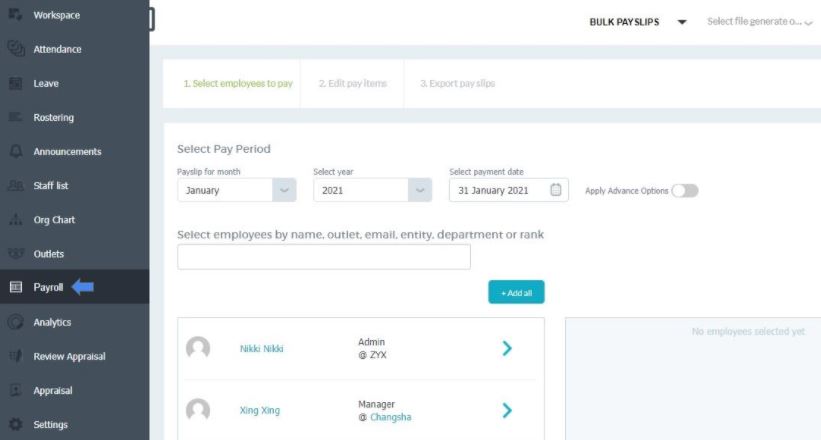This image is a horizontally oriented screenshot capturing a pay period selection screen from a payroll or paycheck management software. On the left side of the screen, there is a dark grey vertical navigation bar featuring various sections. The predominant area of the screen is white, accented with thin, light blue elements, notably in the banner and a small text box at the bottom right corner.

In the top right corner, there is a drop-down menu labeled "Bulk Pay Slips." The main section of the screen, highlighted in white, is titled "Select Employees to Pay." Below this title, a box is provided to choose the pay period, featuring drop-down menus for selecting the month, year, and payment date. 

Further down, there is a text box enabling the user to enter employee details by name, outlet, email, entity, department, or rank. Positioned just below this input field is an "Add All" button.

Within the interface, two employees are listed: Nikki Nikki and Zing Zing. Both are depicted with empty profile pictures. Nikki Nikki is designated as an Admin, while Zing Zing is identified as a Manager. To the right of these employee entries, there is an aqua-colored right arrow.

The design and structure of the screen facilitate the selection and payment processing of employees in an organized manner, ensuring clarity and ease of use.